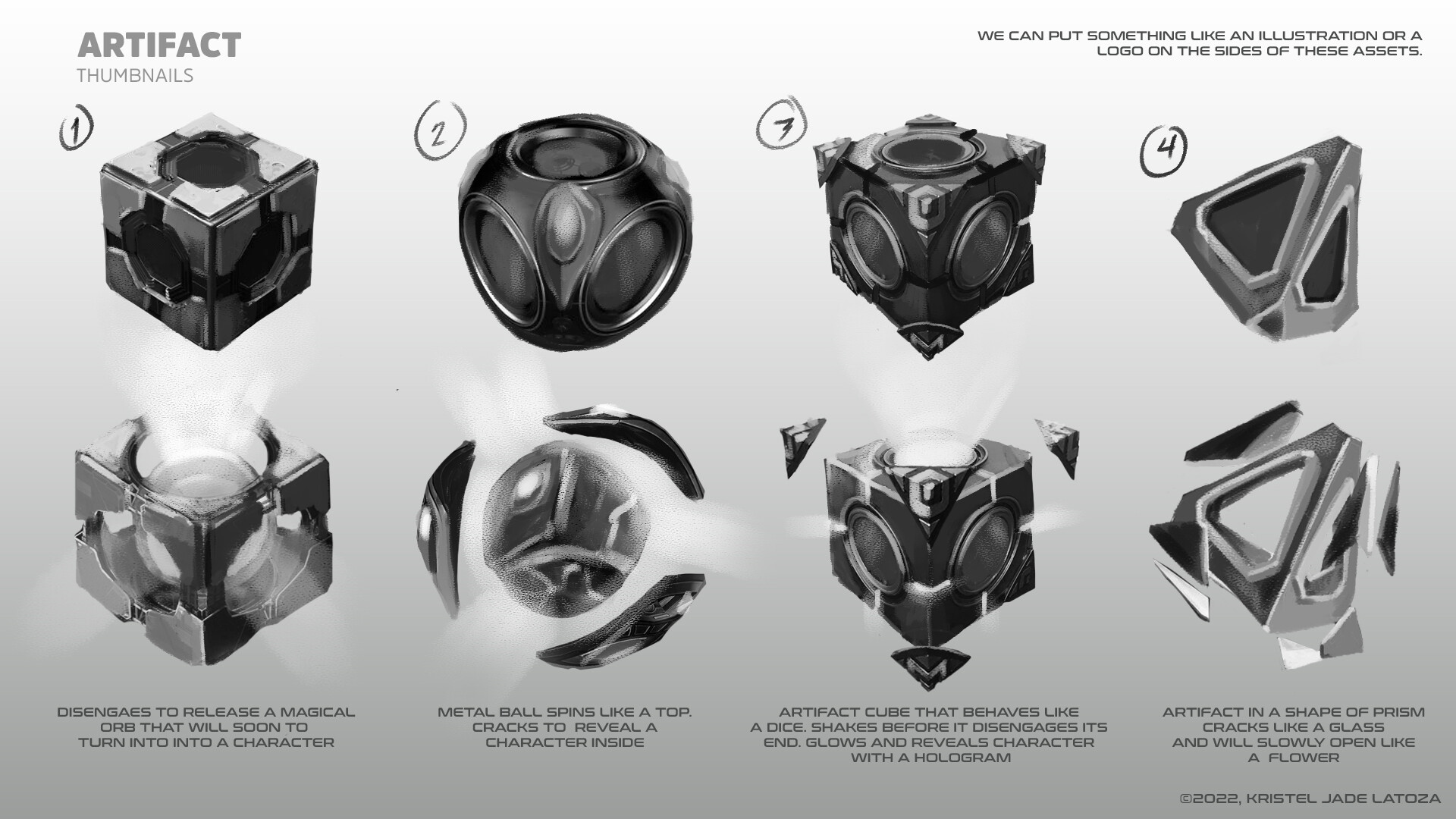The black and white illustration, titled "Artifact Thumbnails," features 8 detailed graphics, arranged in two rows of four, showing various geometric shapes including cubes, spheres, and pyramids. Each shape is uniquely numbered from 1 to 4 within its row. The top left corner of the image contains the heading "Artifact Thumbnails." These shapes, which resemble digital items from a video game, are depicted in both their closed and expanded forms, highlighting their intricate, sci-fi design where sections disengage and expand outward. Descriptions next to each shape reveal their functionalities: a magical orb that transforms into a character, a spinning metal ball that cracks to reveal a character inside, a dice-like cube that glows and projects a hologram, and a prism that slowly opens like a flower. The text on the image is designed to look handwritten, suggesting that these graphics might be customizable stock images or products for sale.